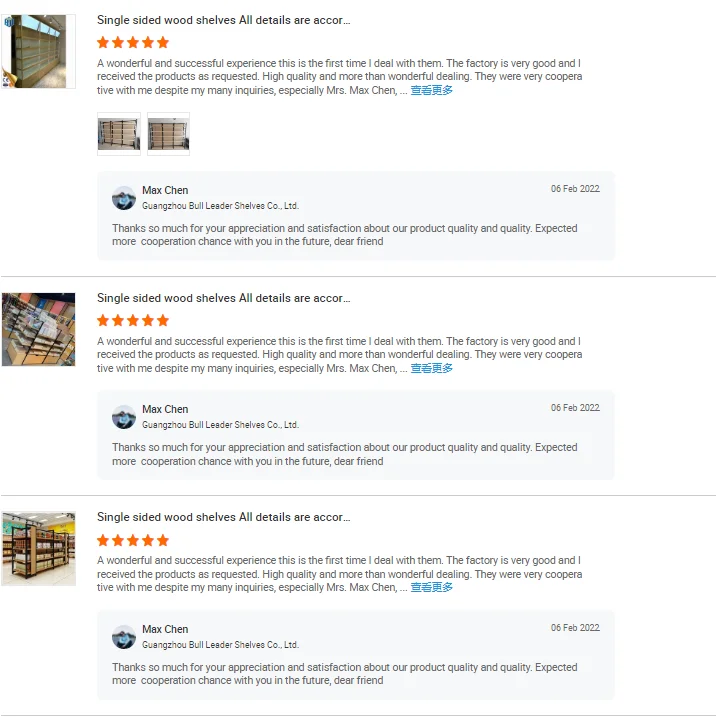The image portrays a listing from a website, focusing on a product titled "Single-Sided Wood Shelves." Notably, all product details are abbreviated as "ACCOR..." due to truncation. Below the listing, there's a user comment from Max Chen, who is identified as being affiliated with "KwanZeguBowLeaderShelvesCO.ltd". His comment, dated February 6, 2022, is set against a light gray background in black text. Max Chen’s comment appears repetitively three times, each instance beneath the listing. The overall background of the depiction, where no images or text exist, is white. The layout additionally includes two small images of the product positioned adjacent to the text.